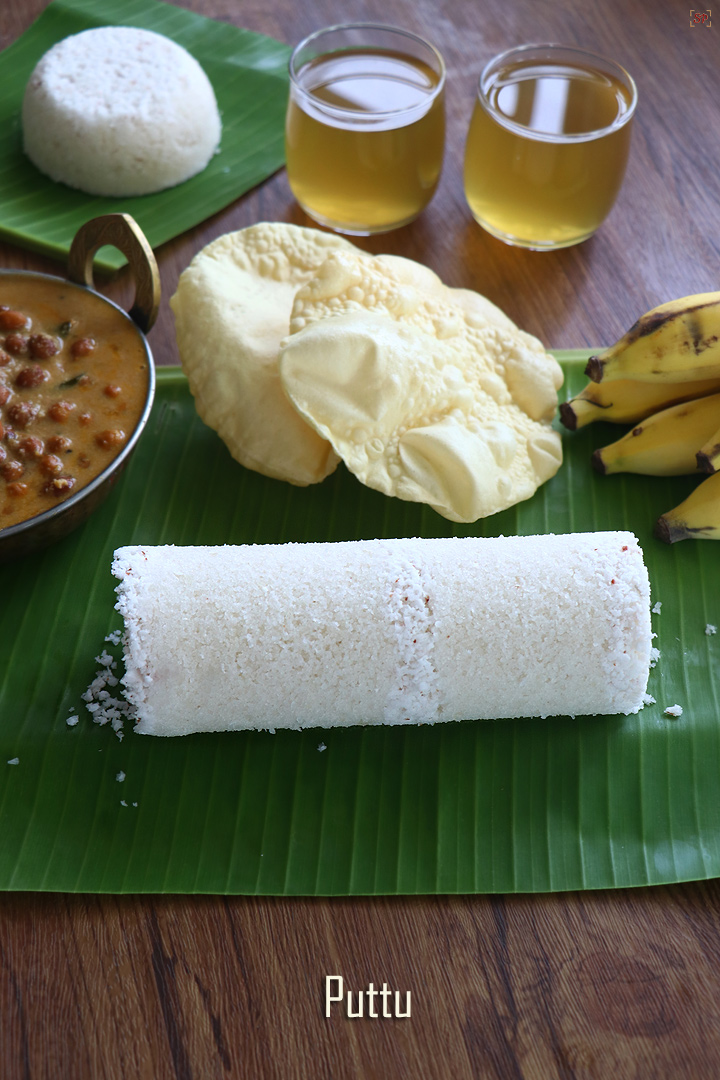This photograph captures a beautifully arranged tabletop scene showcasing an assortment of food items commonly associated with southern Indian cuisine. The table itself is made of golden oak, providing a warm backdrop for the vibrant display. Two banana leaves are prominently featured; the one at the top of the image holds a rectangular section of green leaf topped with a perfect circle of white sticky rice. Positioned above this setup are two short glasses filled with a golden yellow liquid, possibly beer. 

The main attraction in the center features another larger rectangular banana leaf. At the top left corner of this leaf sits a decorative bowl of bean soup, garnished with a brass handle. Mindful details highlight the puffed bread or tortillas, characterized by their bubbly surfaces. Nearby are several ripe bananas or plantains, adding a tropical element to the array. Dominating the center of the image is a long cylinder of white rice, identified at the bottom of the photo as PUTTU, spelled out in text. Puttu is a traditional southern Indian breakfast dish made from rice, typically served either savory or sweet. The careful arrangement and variety of elements evoke a sense of both tradition and culinary artistry.